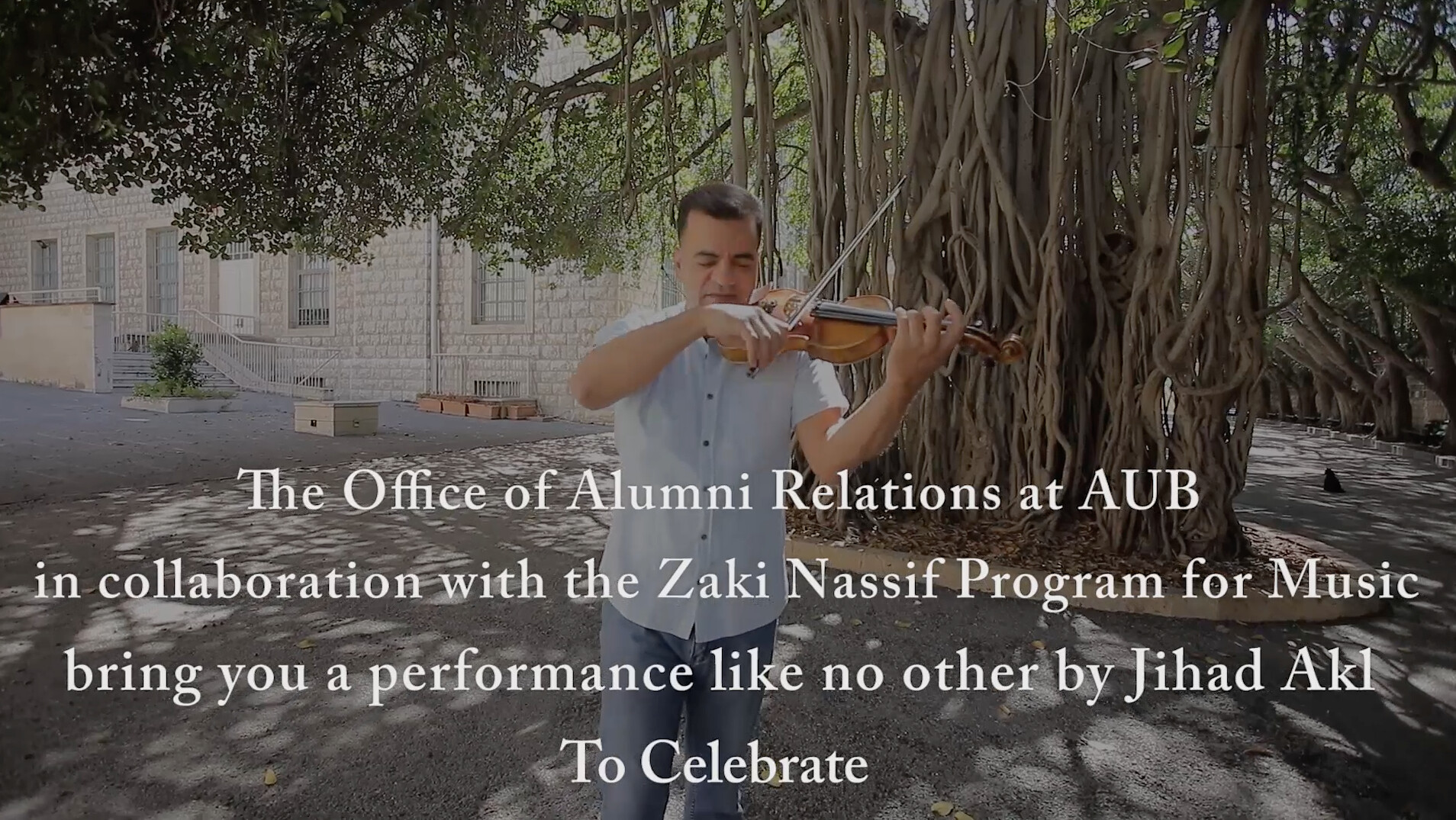This detailed photograph captures a young man, likely in his mid to late 20s, standing outdoors in front of a large, distinctive tree with long, slender, white branches. He is absorbed in playing the violin, holding it with his left arm and strumming with his right. Dressed in a short-sleeve light blue button-down shirt and stonewashed blue jeans, he stands on a cemented area. The backdrop features a building constructed of white bricks with several windows, a stairway, and a patio entrance. The scene is set in daylight, and surrounding trees with abundant leaves add a touch of nature to the environment. White text overlaid at the bottom of the image reads: "The Office of Alumni Relations at AUB, in collaboration with the Zaki Nassif Program for Music, bring you a performance like no other by Jihad Akal to celebrate."